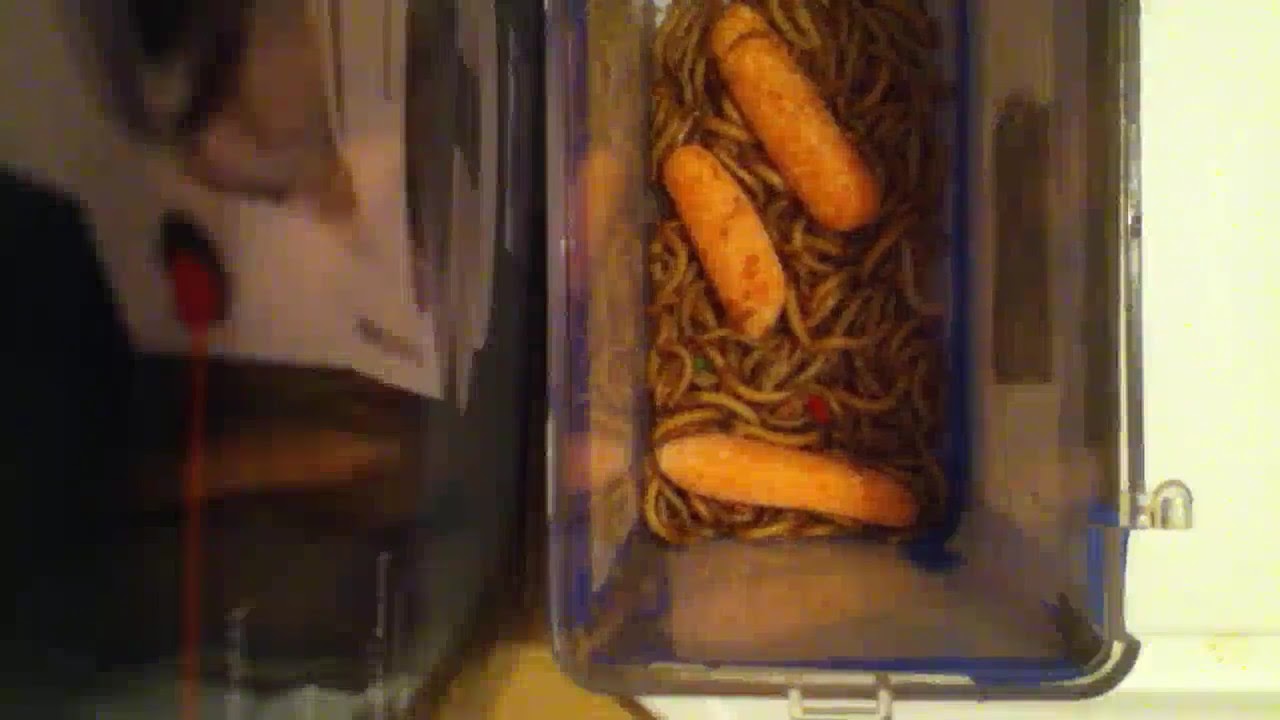The image depicts an indoor scene viewed from a top-down angle. The left side of the photograph is notably blurry, with a faint outline that could be a green rocking chair in the background. The central focus of the image is a clear, deep, plastic container, possibly acrylic, containing food items. The container holds a mix of light brown noodles, likely resembling spaghetti or chow mein. Intermixed with the noodles are red and green pieces, which might be chopped peppers. On top of the noodles lie three elongated, breaded sticks, either resembling fried cheese sticks or possibly baby carrots, although the low quality and compression artifacts of the image render these items ambiguous. The overall scene appears to take place on a table.